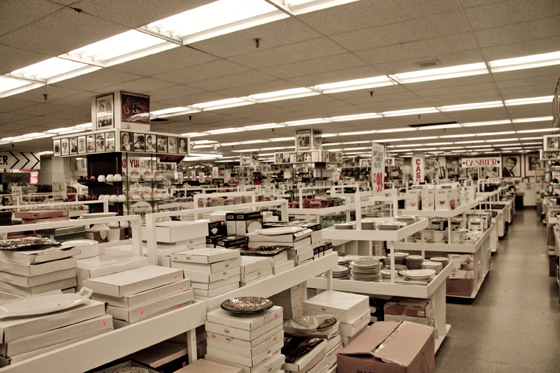This photograph captures the inside of a large department store, likely a home goods store, characterized by traditional white drop ceiling tiles interspersed with rows of fluorescent tube lighting. Dominating the foreground are a series of white, multi-tiered display shelves, each adorned primarily with thin white boxes resembling pizza boxes, topped with various plates and dishes available for sale. Additional shelves in the background support an array of other home interior items such as vases and cups. Prominently visible in the background is a red sign indicating the cashier area. Nearby, a pillar display features photographs of people, adding a touch of human element to the store's interior.